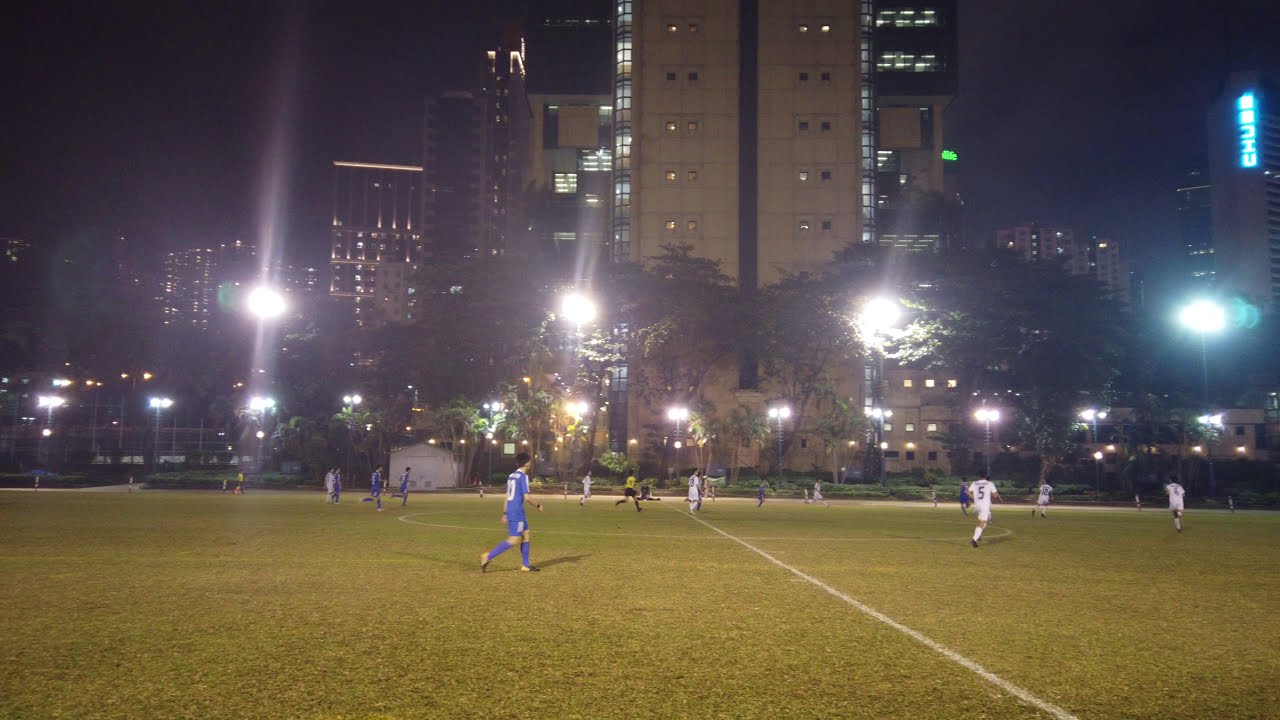This color photograph captures a dynamic nighttime soccer match on a pristine, green grass field marked with white lines. The scene is set under bright overhead stadium lights that cast a crisp illumination on the players and the field, contrasting against the dark night sky. The field is divided into two competing teams: one in blue uniforms with blue socks and the other in white uniforms with white socks. The blue team is positioned on the left side of the field, advancing towards the right, while the white team occupies the right side. The referee stands out in a yellow shirt and black shorts, overseeing the game. In the background, tall multi-storey buildings form an urban cityscape, their windows and the "Chubb" logo on one building glowing brightly in the night. The photograph, taken from a drone, offers a comprehensive and realistic view, showcasing not just the fervor of the game but also the vivid details of the surrounding city life.